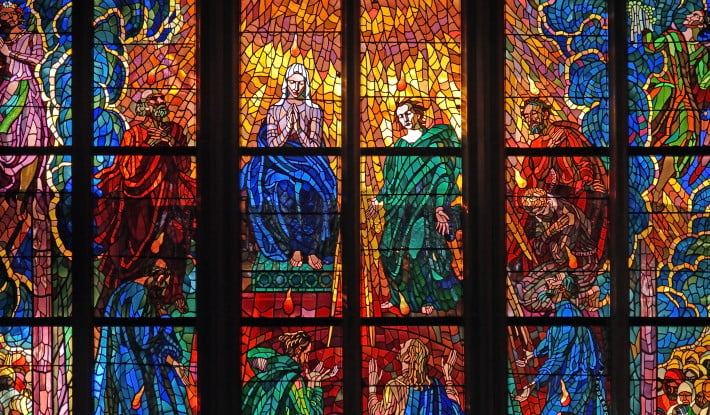This detailed photograph captures the exquisite stained glass windows of a chapel, showcasing an array of vibrant, multi-paneled artistry. Dominated by bright yellows, reds, purples, and pinks, the central sections of the stained glass radiate with the intensity of sunlight, creating a striking focal point. The scene prominently features the Virgin Mary on the third pane, adorned in a white head covering and a blue cloth draped across her lap, with her hands clasped in a prayerful gesture. Surrounding her are several reverent figures, each robed in vibrant hues of red, green, and blue. Some of these figures have their heads bowed or eyes closed, embodying a state of prayer. This vivid tapestry of holy figures and abstract forms is bathed in a harmonious blend of colors, ranging from the bright blues, greens, and reds of the robes to the lighter and darker shades of orange and red in the background, depicting a richly spiritual scene steeped in religious reverence.